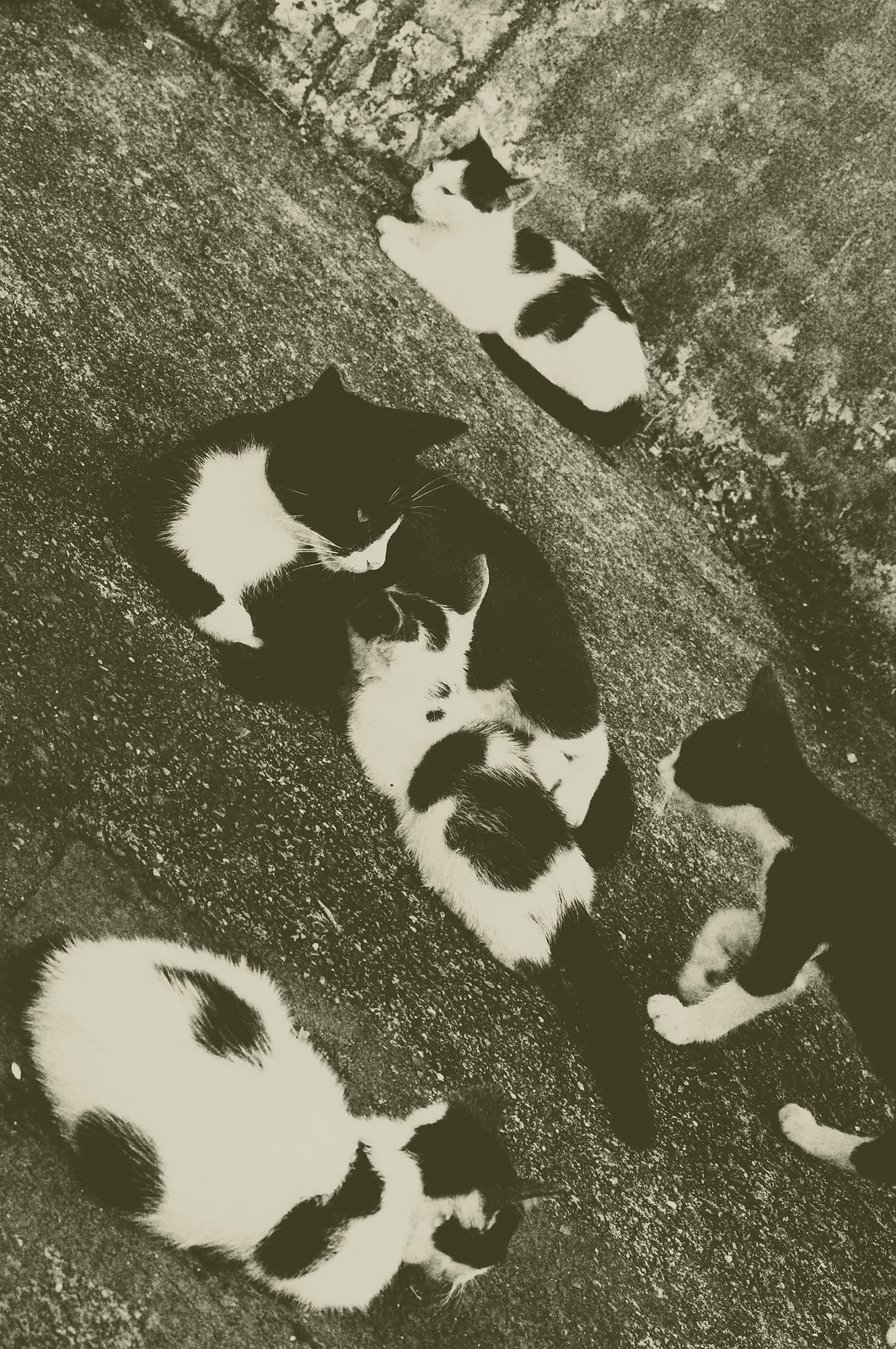This is a vertical black-and-white photograph of five black and white tuxedo cats, slightly tilted, making the ground run diagonally from the top left to the bottom right. They are situated on a hard gray background with a somewhat grimy wall behind them. At the center of the image is the largest cat, predominantly black with a white chest, which appears to be nursing a smaller kitten. This nursing kitten is primarily white with distinct black spots on its head, back, and a black tail. Close to them, another cat is partially obscured, tucked under the large cat, sporting black splotches on its head, a white face, and additional black splotches on its back. In the foreground, a smaller kitten is visible, characterized by black splotches on its back, black ears, and the black top of its head. On the right side, a tuxedo kitten is positioned in profile, featuring white feet, a white nose, and chin, against its primarily black coat. The tilted perspective gives this detailed composition a dynamic quality, bringing attention to the interactions and distinct patterns of each cat.